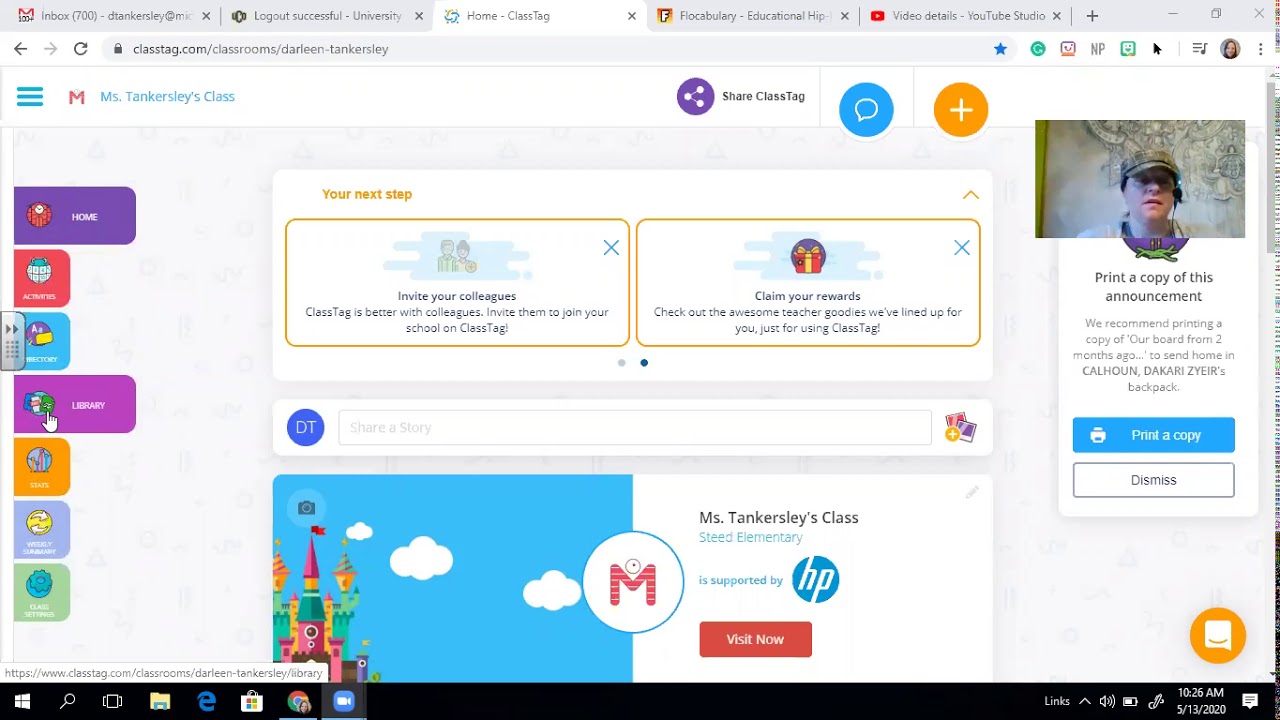The image displays a computer screen showcasing Ms. Darlene Tankersley's class website on ClassTag. The browser has numerous open tabs, and the current one selected is labeled "Home" with the URL "classtag.com classrooms Darlene Tankersley." 

On the left side of the screen, a vertical sidebar contains a variety of clickable tabs, with one labeled "Library" highlighted by a hand-shaped cursor. The banner at the top of the page prominently features "Tankersley," accompanied by a blue speech bubble icon for class communication.

An announcement is visible at the top of the page, featuring an image of an individual and text suggesting printing a copy of the board from two months ago to place in Calhoun Dakari Zier's backpack, with options to print or dismiss the announcement.

In the center of the screen, a section titled "Your Next Steps" provides instructions to invite colleagues or claim records. Below this section, a search bar is available for easy navigation. The bottom area of the page indicates that Ms. Tankersley's class is supported by Hewlett-Packard, highlighting the website's role in facilitating online work for the class.